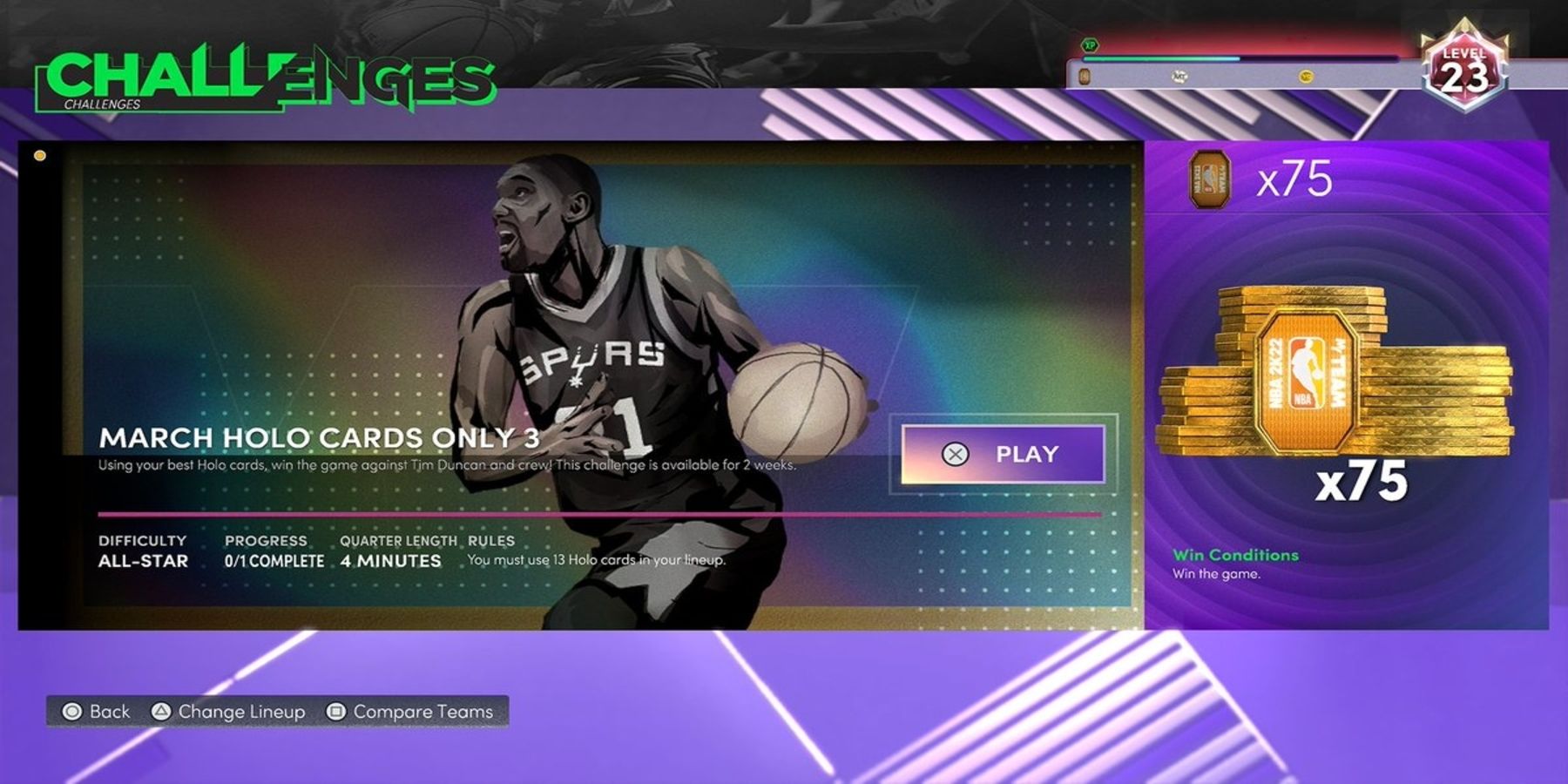The image appears to be a screenshot from a basketball-themed video game interface. The primary background color near the bottom is a rich purple, interspersed with horizontal and diagonal white lines. In the lower-left corner, there is a long gray rectangle featuring the options: "Back," "Change Lineup," and "Compare Teams," indicating in-game functionality.

Dominating the left side of the image is a dynamic picture of a man in a Spurs basketball jersey displaying the number 1. He is captured in a moment of intensity, with his mouth open and seemingly preparing to make an exciting move, possibly charging forward. He holds a basketball in one hand. 

Below his image, to the left, there is text that reads "March Holo Cards Only." To the right of this text is an option button labeled "Play," accompanied by a small X icon for closing or canceling. Adjacent to the play option are three clusters of stacked gold coins, with "X 75" written underneath the coin icons, likely indicating in-game currency or rewards.

In the upper left corner, the word "Challenges" is displayed prominently in bright green text, with a black diagonal line striking through the first 'E.' Finally, in the upper right corner, there is a diamond-shaped icon containing the number 23, possibly representing a score, rank, or another game element.